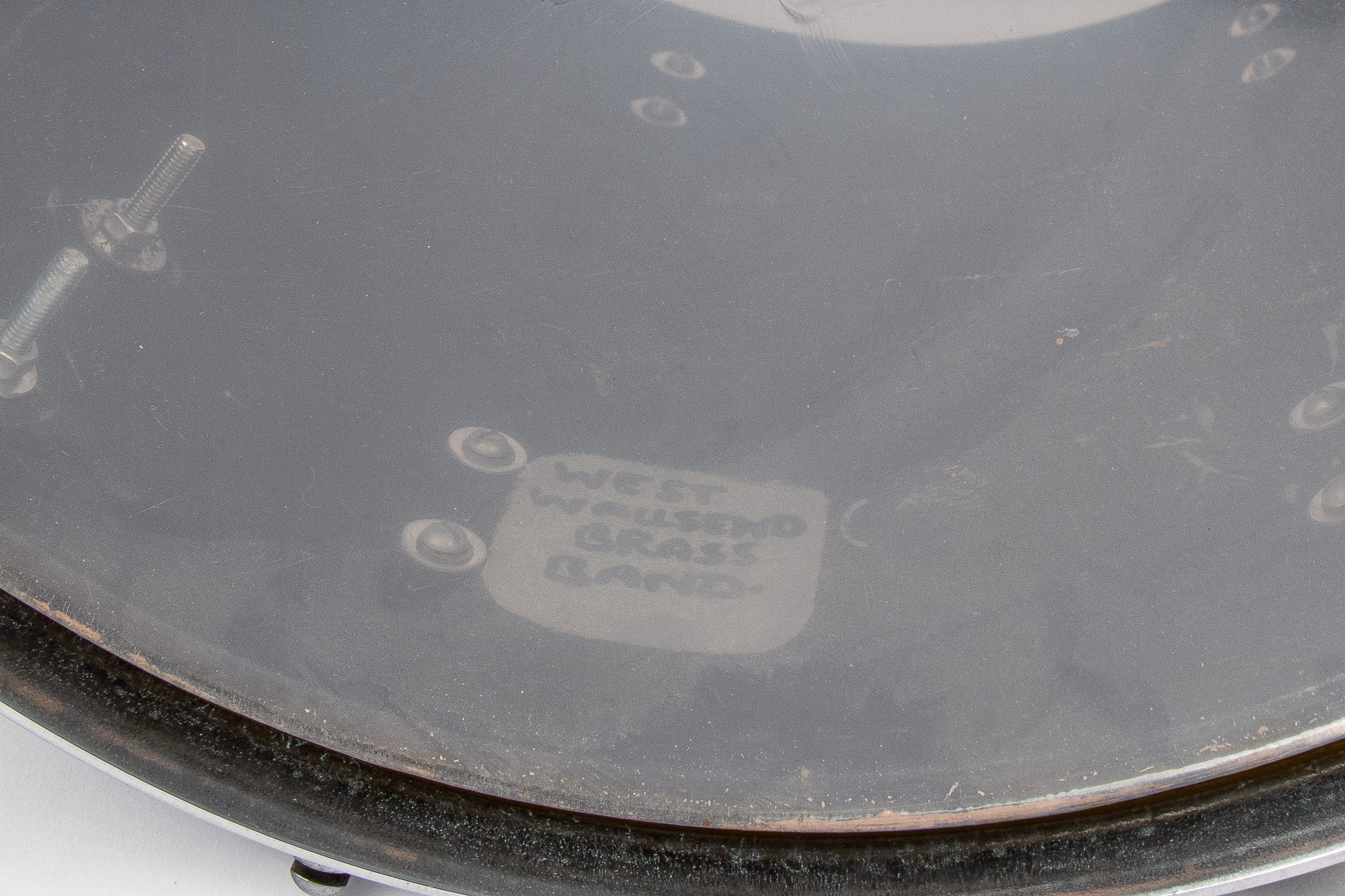The image is a detailed close-up of a drum's translucent and scuffed drumhead, part of a larger drum kit, likely used in performances by stepping on a pedal to produce sound. The photograph, capturing a dusty and old-looking drum, highlights the text "West Walzend Brass Band" in black on a white sticker. The drum's surface appears gray and powdery, with visible screws and bolts around its edge, some with a hint of rust. The overall monochromatic tones, combined with the industrial look of the connections and divots, suggest it's an integral part of a well-used drum in a brass band setup.